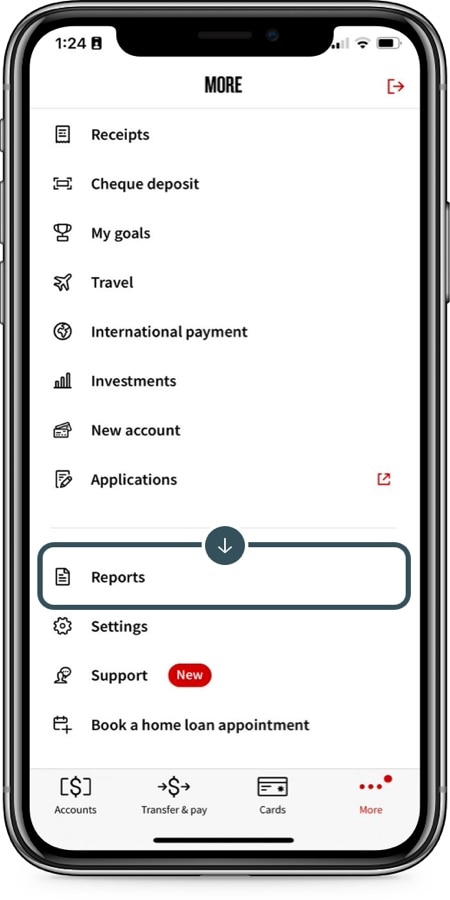In this image, an iPhone displays an app interface named "More." The app's background is primarily white with black text for various menu options. At the top of the screen, "More" is prominently displayed, indicating the app's name. Below this header, the main menu lists several options: "Receipts," "Check Deposit," "My Goals," "Travel," "International Payment," "Investments," "New Account," "Applications," and "Reports," which is currently highlighted and features a down arrow suggesting further interaction. Following "Reports," the options continue with "Settings," "Support" (marked as a new feature), and "Book a Home Loan Appointment."

At the bottom navigation bar of the app, there are four buttons labeled "Accounts," "Transfer and Pay," "Car," and "More."

In the top right corner of the phone screen, typical device indicators are visible, including the battery level, Wi-Fi signal, and cellular signal bars, affirming that it's an iPhone. On the top left corner, the time reads 1:24.

This app appears to offer a comprehensive suite of financial and organizational tools, helping users manage receipts, deposits, goals, travel plans, international payments, investments, account setups, applications, and more, thereby aiding in personal growth and efficient tracking.